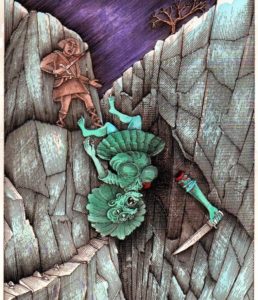In this detailed cartoon-style image, two characters are set against a dramatic rocky landscape with a dusky sky tinged with hues of purple and blue. To the left, perched on the edge of a towering cliff, stands a warrior-like figure predominantly clad in brown. This character, identifiable as a man due to his short, blunt-cut hair reaching his ears, wields a white sword in his right hand. His attire and stance embody a battle-ready presence.

To the right, a female character, distinctively green from head to toe, including her skirt and shirt, is depicted falling from the rocky precipice. She has a large headpiece and is barefoot, with flowing big hair and discernible breasts, emphasizing her femininity. In a shocking visual twist, her left arm has been severed and is separately falling alongside her, gripping a knife in its hand. Red marks illustrate the bloody wound where her arm was cut off. The rocky terrain is detailed with gray, cracked stones shaded in darker tones, enhancing the scene's intensity. The silhouettes of trees are also visible in the background, contributing to the overall atmosphere of an intense and perilous moment captured in a mix of animation and painting styles.